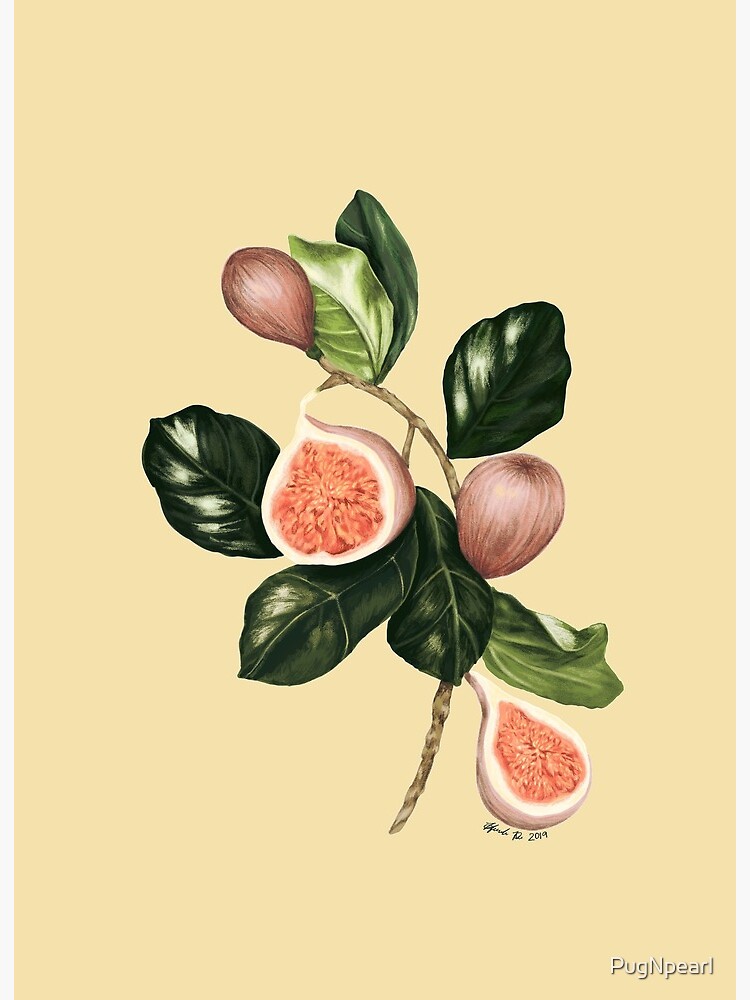This vertical hand-drawn image, set against a pale apricot yellow background, is watermarked with the small, white font text "Pug and Pearl" in the bottom right corner. The central focus of the artwork is a branch showcasing six deep green leaves, artfully highlighted with varying shades of green. Prominently featured are four fig fruits: two intact and two cut in half, revealing a spongy pink fruit-like interior. The figs display a harmonious palette of light pink, orange, mauve, and tan-brown hues.